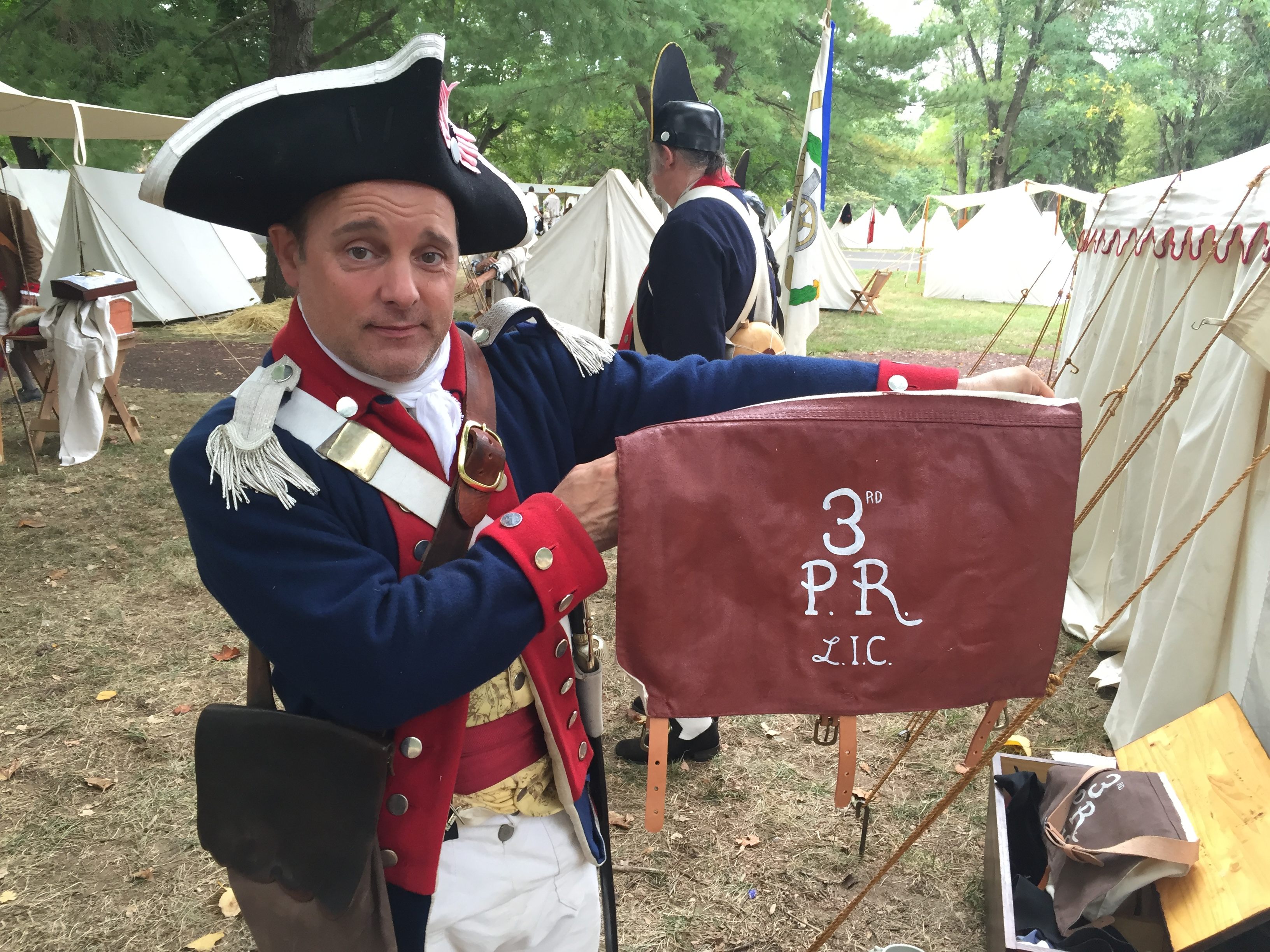The color photograph captures an outdoor scene featuring two men dressed in Revolutionary War-era military uniforms. Central in the image, a man stands facing the camera, adorned in a dark blue coat with red sleeves and silver buttons. He wears a white scarf around his neck and a tri-corner hat that is black with a white border. His right shoulder bears white tassels and a white strap that likely belongs to a backpack, while a brown flat bag hangs over one shoulder. Holding a maroon rectangular piece of cloth that reads "3rd PR LIC" with both hands, he stands on greenish-brown grass, surrounded by numerous white tents and trees in the background. Another man, clad in a similar uniform, stands slightly behind him, turned to the left. A brown bag sits inside a box at the right corner of the photograph.